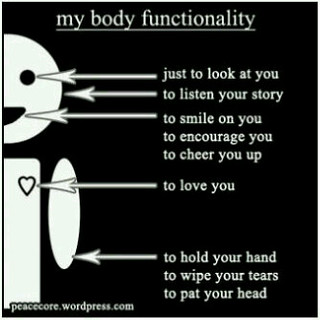The image features a black background with the text "my body functionality" written in an underlined white font at the top. On the left side of the image, there is a white stick figure-like robot creature with a square body, a floaty oval arm, and a cartoon heart on its chest. The figure is smiling, though only half of its body is visible. Arrows connect various parts of the figure to corresponding descriptions in white text on the right side. These descriptions detail the figure's functions: "just to look at you" pointing to the eye, "to listen to your story" pointing to the cheek, "to smile on you, to encourage you, to cheer you up" pointing to the mouth, "to love you" pointing to the heart, and "to hold your hand, to wipe your tears, to pat your head" pointing to the hand. The image ends with a citation to peacecore.wordpress.com.